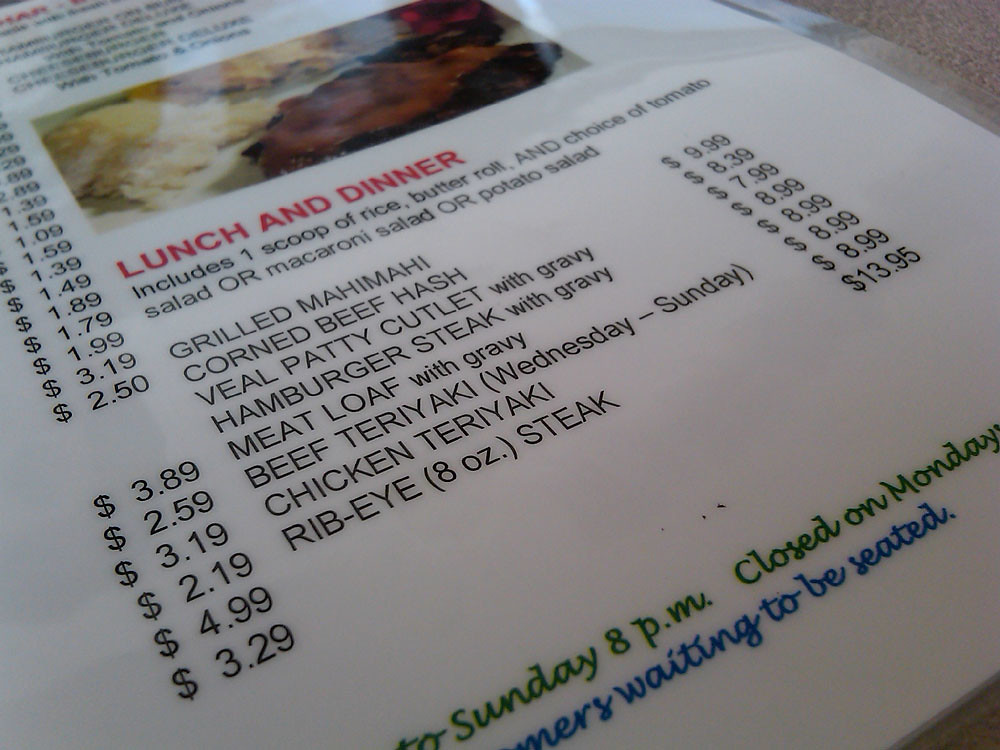The photograph captures a menu placed on a flat surface, taken from an angle that creates a perspective leading the bottom edge of the menu towards the bottom right corner of the image. The left side of the menu lists various prices, while the top right features additional food items. 

At the very top of the menu, there is an image of some food, although it's somewhat blurry and hard to distinguish. Below this image is a section titled "Lunch and Dinner" in bold red text. Following this, the menu states that each meal includes one scoop of rice, a butter roll, and a choice of tomato salad, macaroni salad, or potato salad.

The listed dishes under this section, along with their prices, are as follows:
- Grilled Mahi-Mahi: $9.99
- Corned Beef Hash: $8.39
- Veal Patty Cutlet with Gravy: $7.99
- Hamburger Steak with Gravy: $8.99
- Meatloaf with Gravy: $8.99
- Beef Teriyaki (available Wednesday-Sunday): $8.99
- Chicken Teriyaki: $8.99
- Rib Eye, Eight-Ounce Steak: $13.95

Near the bottom of the menu, there is text in a cursive font detailing the hours of operation. It reads: "Tuesday to Sunday, 8 p.m." and "Closed on Mondays." Additionally, there’s a note in blue cursive stating, "Please wait to be seated," and above the "Closed on Mondays" notice is text in green cursive.